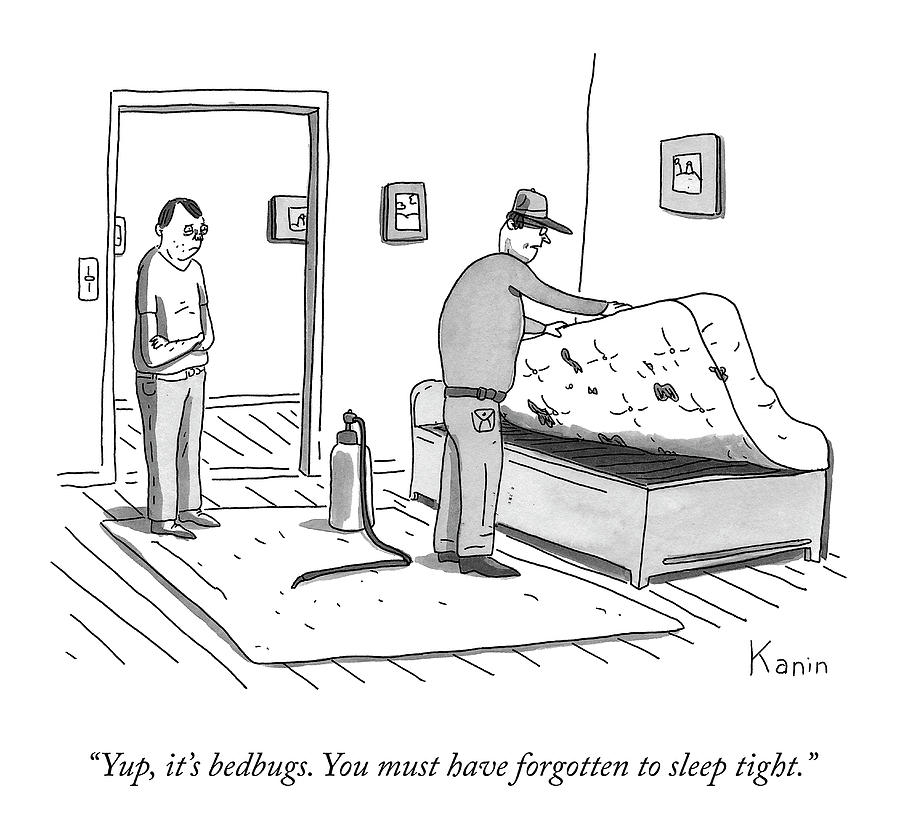This black-and-white cartoon illustration captures a humorous yet unfortunate scene with meticulous detail. Centered within a sparsely decorated bedroom featuring a wooden floor and a rug, an exterminator dressed in a uniform and baseball cap lifts up a mattress to reveal bedbugs underneath. The spray bottle with a hose beside him emphasizes the nature of his work. Nearby stands the distressed homeowner, clad in a t-shirt, bare arms, slacks, and shoes, with his arms crossed and a baffled expression on his face. The room is completed by a few pictures hanging above the bed and seen faintly through the doorway in the upper left corner, next to which there is a light switch. The bottom of the image contains a cheeky caption in italicized black text: "Yup, it's bedbugs. You must have forgotten to sleep tight," adding a touch of satire to the situation. The cartoon is artistically signed "KANIN" in the bottom right corner, providing a personal touch to the piece.